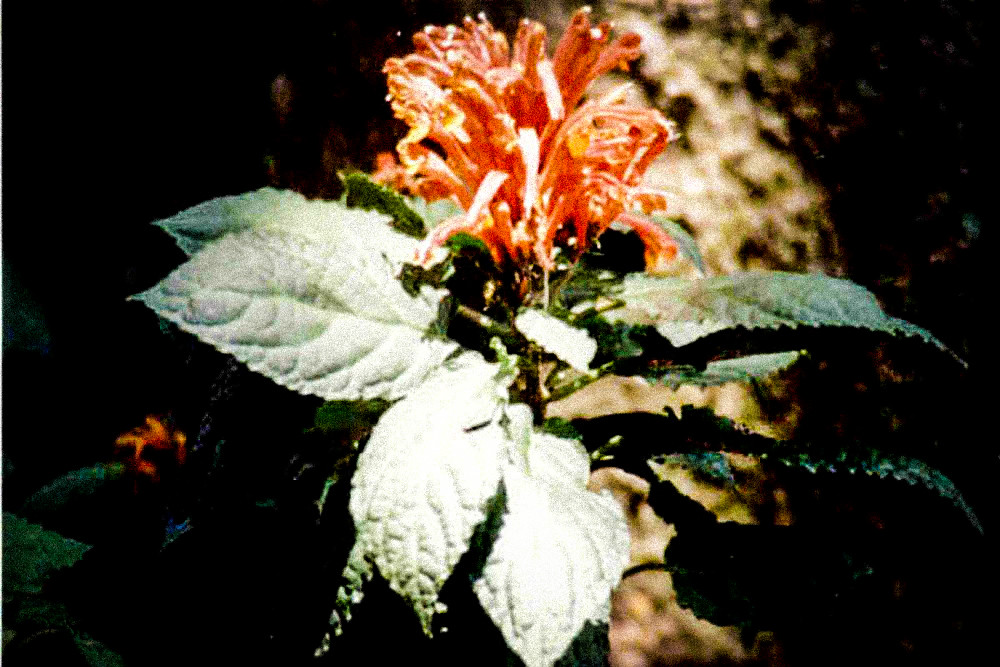The photograph showcases a vibrant, reddish-orangish flower with numerous thin petals reminiscent of shredded carrots, arcing upwards. It is surrounded by jagged, shiny green leaves, numbering about 8 to 10, although the intense lighting from the camera flash gives the leaves a yellowish sheen. The background is predominantly dark, with a hint of a garden setting, possibly containing more faintly visible flowers. Directly behind the bloom and leaves, there is a blurry, brownish area that might be a rock, adding a subtle textural contrast. While some mention of people in the background is less clear, the overall impression remains a brightly illuminated plant set against a predominantly dark, indistinct backdrop, highlighting the flower's vivid colors and detailed structure.